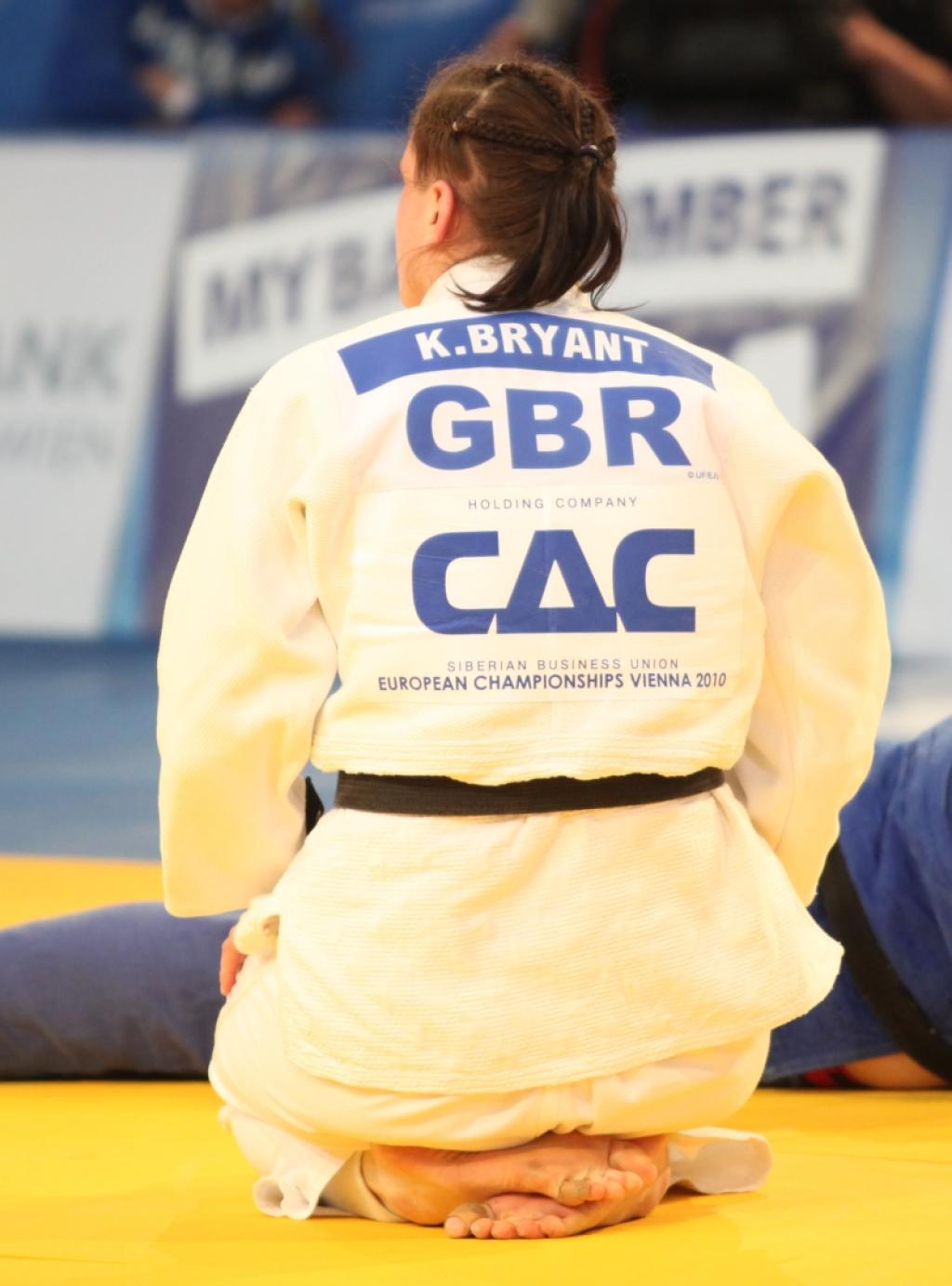This realistic photograph captures a scene likely from a competitive event, possibly the Olympics or a similar competition. The image centers on two individuals positioned on a brown gym mat, suggesting an indoor sports setting. The focal point is a person in the middle, adorned in a long white robe, sitting cross-legged on their knees with their bandaged feet visible. The back of the robe features blue text that reads "GBR Holding Company, CAC, Siberian Business Union, European Championships, Vienna, 2010," and above this, a blue rectangle with white writing that says "K. Bryant." This individual, a white person, has long hair styled in a braided ponytail. In front of them lies another person dressed in blue attire, with some skin peeking through the side. The background is filled with various banners advertising different companies, adding to the competitive atmosphere of the scene.